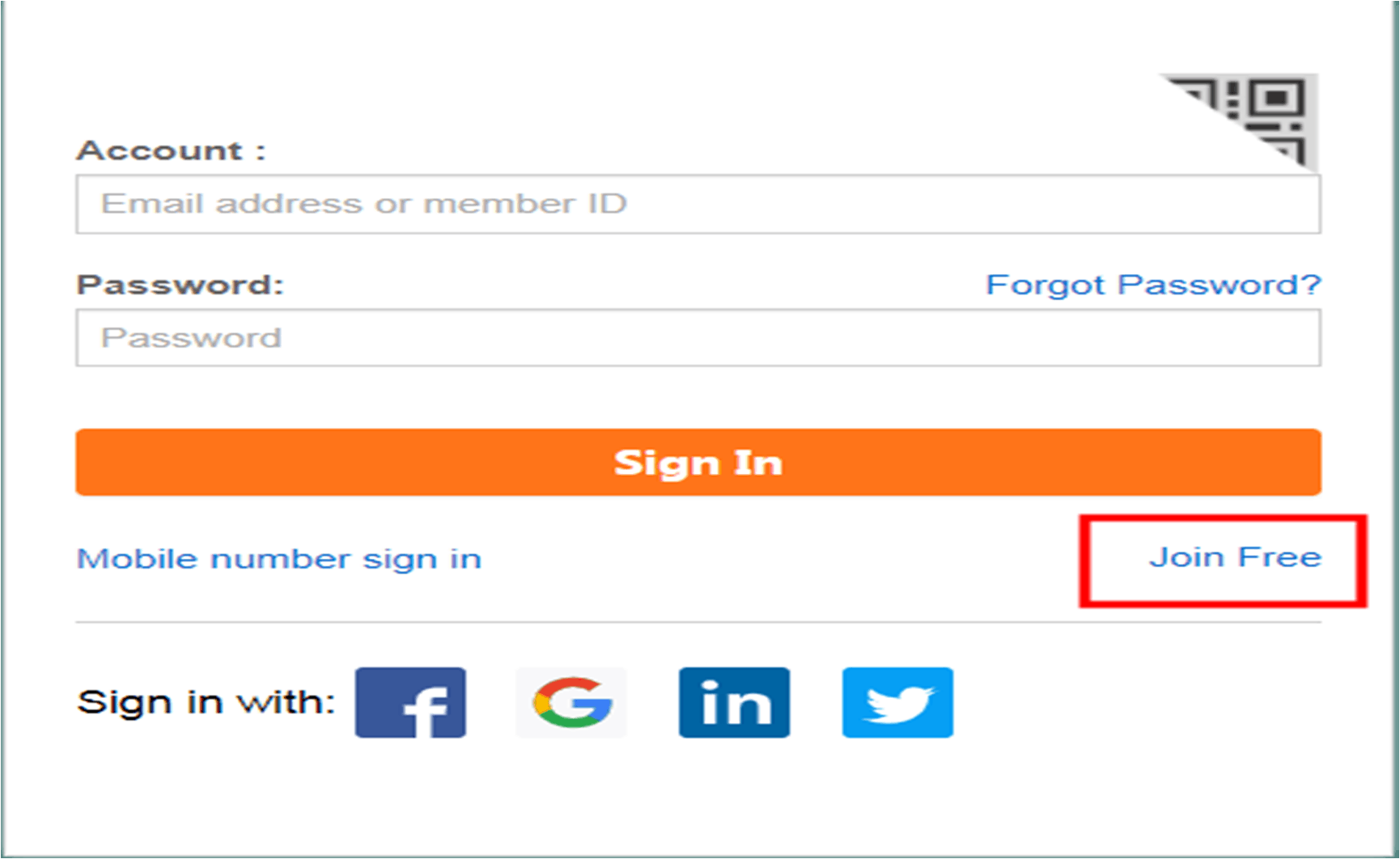The image depicts a login page set against a white background. The top section is missing a header, and there is a partially ripped QR code on the right-hand side, diagonally torn. Below the absent header, there is a text label "Account" followed by a box for entering either an email address or member ID. Beneath this, there's another label that reads "Password" accompanied by a white box to input the password. To the right of the password box, there is a clickable "Forgot password?" link displayed in blue text with a question mark.

At the bottom of the input fields, there is an orange bar with white text that reads "Sign In." Below this orange sign-in button, there is another option in blue text that says "Sign in with mobile number," and a contrasting "Join Free" button contained within a red-bordered box with a white background.

At the lower section of the page, the image shows alternative sign-in options with different platforms: Facebook, Google (represented by a standalone 'G' without a surrounding box), LinkedIn, and Twitter. Each of these platform options is distinguished by their respective colors and logos.

The entire layout is enclosed within a very thin gray line, giving structure to the website’s design.